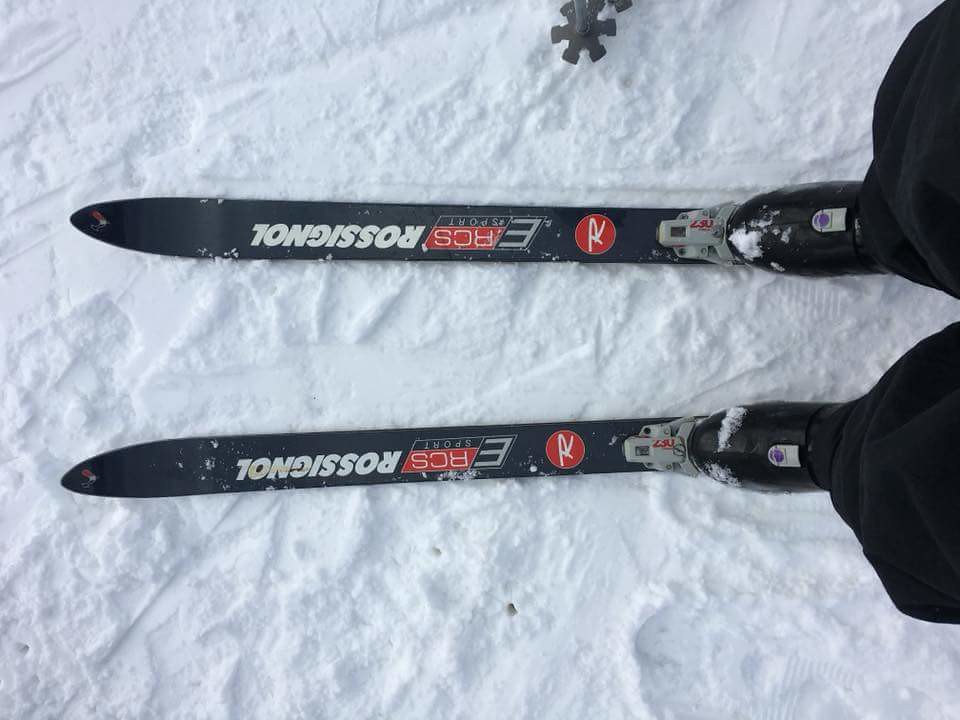This photograph offers a detailed view from the perspective of the skier, showcasing a pair of black Rossignol ERCS Sport skis against a snowy surface. The image is taken at an angle, displaying the skier’s feet on the right, clad in black boots and black pants, with the ski tips pointing to the left. Visible gray bindings secure the boots to the skis, which also feature a distinctive white "Rossignol" logo, upside down in the shot. Above the bindings, a red circle with a white "R" stands out. Additionally, ski poles are visible at the top of the image. The snow on the ground appears to be well-trodden rather than freshly fallen.